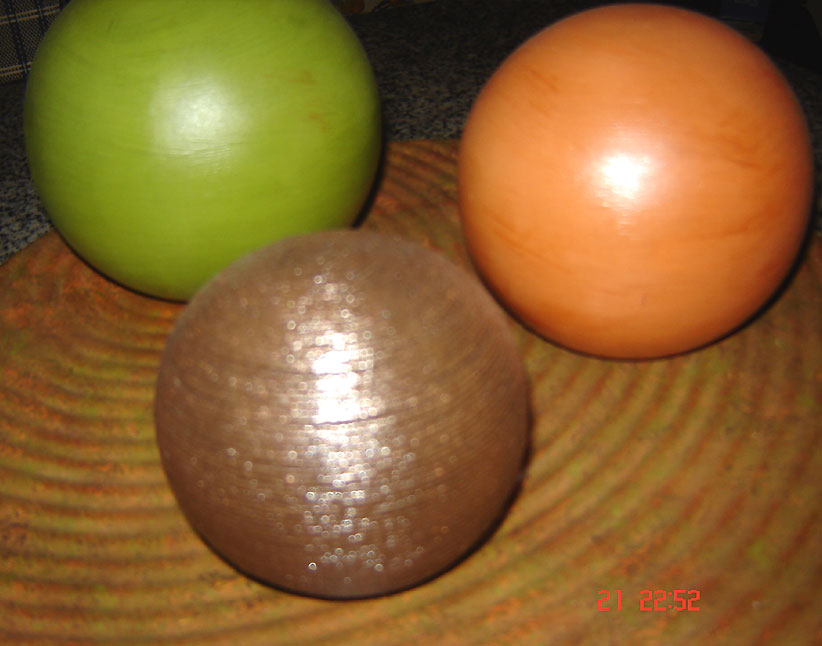The image shows a slightly wider-than-tall composition featuring three balls resting on a wooden surface with concentric circular rings. The wooden surface, likely a tray or mat, exhibits an intricate pattern of light and dark browns. A lime green ball with brown spots sits in the upper left corner, partially concealing the center of the rings. Below and to the right is a darker, copper brown ball with a rippled texture, while an orange ball with darker spots sits above and to the right. A gray and black marbly granite-like countertop can be seen at the top left and top of the image, forming the background. In the lower right corner, the numbers "21 2252" are displayed in red text, possibly indicating a time and date. The light source appears to be coming predominantly from the front, casting reflections on the balls.